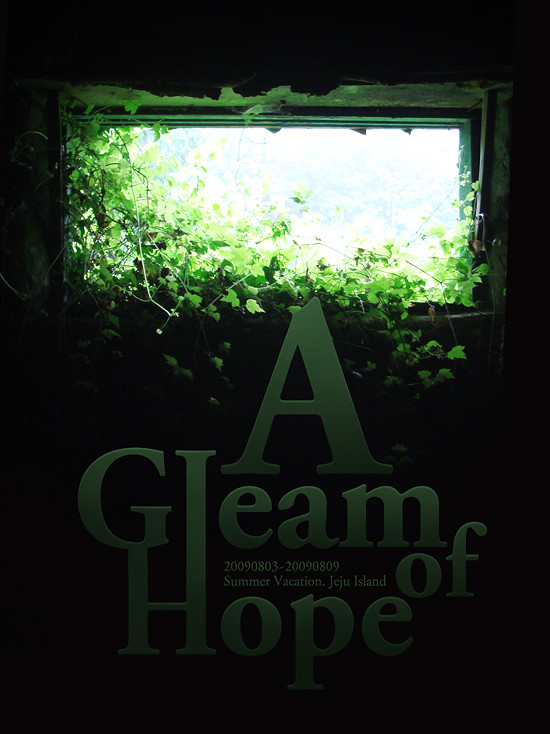The image features a dark poster with a black background. Dominating the scene is a rectangular window located near the top left corner of the wall. The window's width is greater than its height, and it appears to open to the outside, where light is visible. Around the window, lush green vines with three-sectioned leaves crawl and seep into the frame, denser in some areas than others. Distinctly, some frost or ice-like texture is visible near the top of the window. Below the window runs a line of green text, although hard to read due to the dark surroundings. The text reads "A Gleam of Hope" with the dates "2009-08-03 to 2009-08-09," followed by "Summer Vacation, Jeju Island."